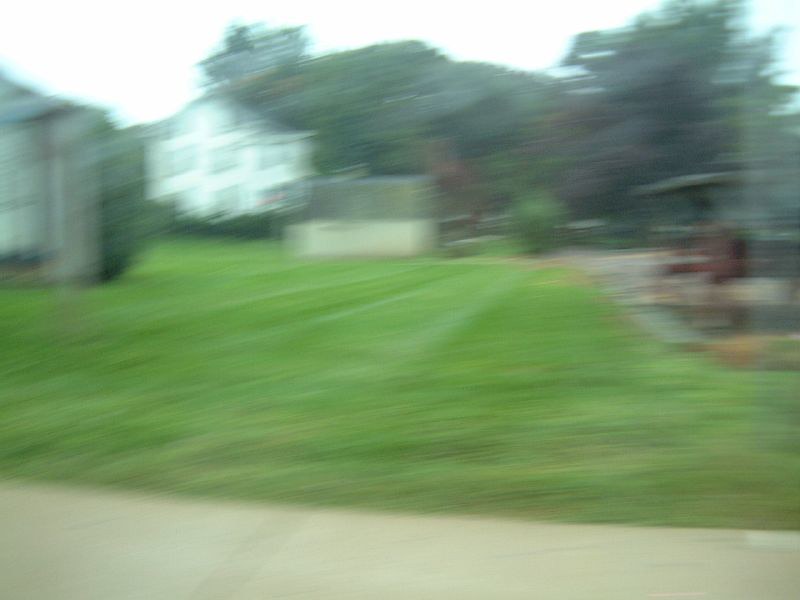A highly unfocused image depicting a grassy lawn. The photograph suffers from significant blurriness, making it difficult to discern any specific details or features of the lawn. The greenery is still somewhat identifiable, though the overall image lacks clarity.